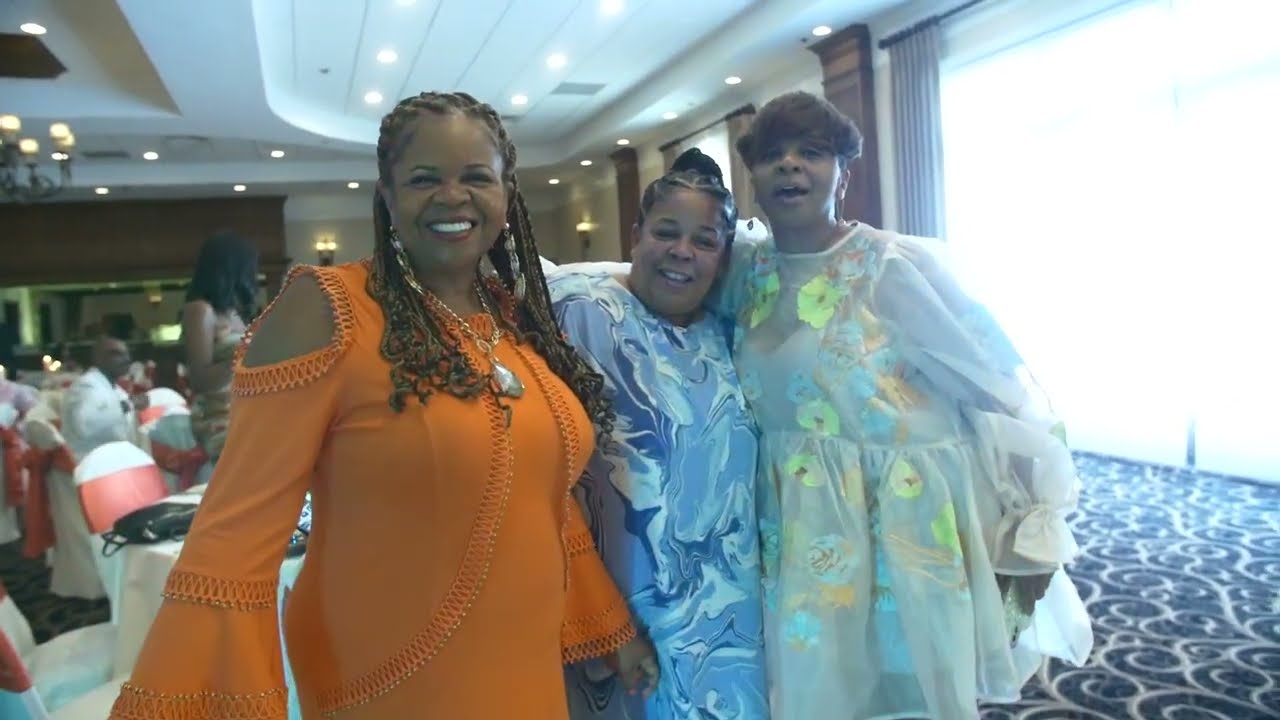This photograph captures a joyful moment at a likely festive event, possibly a wedding, held in a spacious indoor dining hall. Centered in the image are three distinguished Black women, all smiling warmly and directly at the camera. Their attire is notably colorful and elegant: the woman on the left wears an orange dress with oversized wrist cuffs, the middle woman dons a blue dress featuring a tie-dye or marble-like pattern, and the woman on the right graces the scene in a white dress adorned with yellow floral prints. They appear to be close in age, with the left and middle woman possibly in their 40s, and the right one seemingly in her early 20s. The trio stands arm in arm, exuding a sense of camaraderie and affection. In the background, the hall is filled with circular tables dressed in white tablecloths, surrounded by chairs, and occupied by other well-dressed attendees. The room is illuminated by overhead lighting set against a white ceiling, and light also streams through a large window or gate on the right side of the frame.